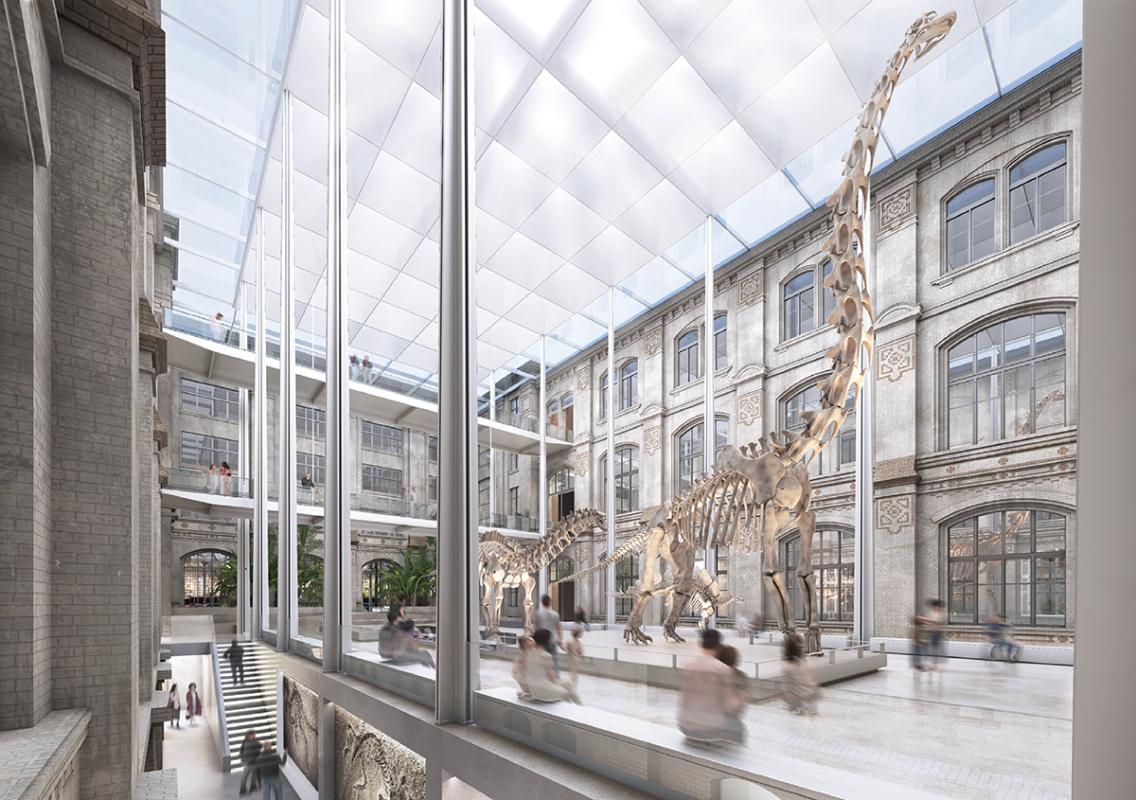This image depicts the interior of a museum featuring a time-lapse photograph showcasing a large dinosaur skeleton, identified as a Brontosaurus, with a smaller dinosaur skeleton behind it. The photo, taken through a series of clear windows, highlights the blurred, translucent silhouettes of people moving around, indicating the passage of time. The museum's layout includes upper levels and staircases, allowing visitors to view the dinosaur exhibits from various heights. The environment is characterized by a clear ceiling, wooden floors, and surrounding structures, which remain consistent even as the people appear in motion. The dinosaur skeletons, prominently displayed, are the focal points amid the dynamic, fast-paced atmosphere of the museum.